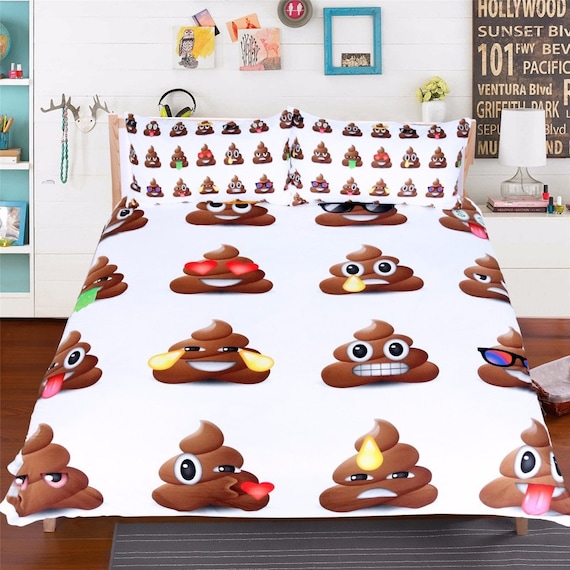The image depicts a digitally staged children's bedroom with a playful and colorful theme, set against a white backdrop. Central to the scene is a white comforter adorned with various poop emojis displaying a range of expressions, including hearts for eyes, blowing a kiss, sticking out a tongue, wearing sunglasses, smiling, throwing up, crying tears of joy, and sweating. This pattern runs throughout the bedspread and shams, organized in rows of four repeating icons. The bed is placed on a gray carpet over a wooden floor, and is accompanied by a sign listing various streets in Los Angeles, such as Hollywood, Sunset Boulevard, and Mulholland Drive. The left side of the room features a bookshelf with white shelves and a blue backing, while to the right, a side dresser holds nail polish and has antlers adorned with necklaces. Additionally, there are paintings or artwork on the walls and a pair of headphones placed right behind the bed.